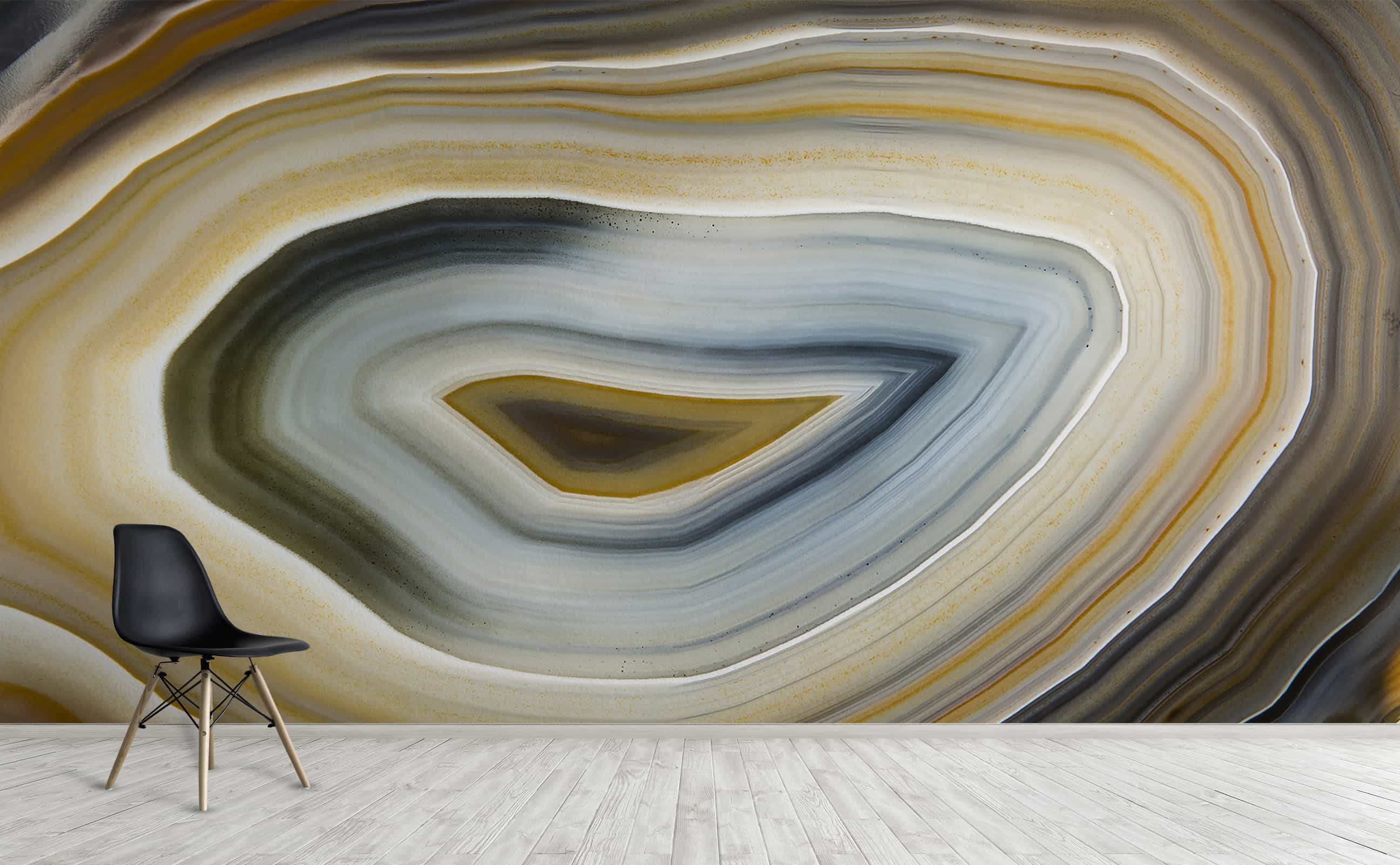The photograph, captured indoors, features a detailed and vibrant setting. The bottom half-inch reveals a polished, whitewashed wooden floor with vertical planks. In the foreground, to the left, sits a modern, minimalistic black chair with four brown wooden legs, contrasting starkly with the floor.

Dominating the background, a large, painted wall commands attention. This wall art mimics the intricate, layered patterns of a geode or petrified wood cross-section. At the center of the mural, there's a dark brown diamond-shaped figure, which radiates outward in a series of concentric rings. These rings transition from dark brown to lighter coffee-colored cream, interspersed with bands of blue. The blue bands range from light to dark, adding depth and texture to the design. The outermost layers feature darker browns, completing the rich, earthly palette of the geode-like painting.

The combination of the polished wooden floor, the sleek black chair, and the striking wall art creates a harmonious blend of modern minimalism and natural inspiration within the large room.